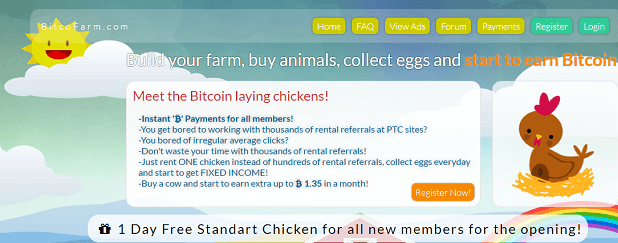This is a screenshot of the webpage bitcofarm.com, as indicated in the top left corner. The background features a charming farm scene with a vibrant sun partially obscured by a cloud and a colorful rainbow. The page promotes its unique proposition with the headline: "Build your farm, buy animals, collect eggs, and start to earn Bitcoin." Below this, it states: "Meet the Bitcoin laying chickens. Instant Bitcoin symbol payments for all members." 

It addresses user concerns candidly: "Bored of working with thousands of rental referrals at PT sites? Tired of irregular average clicks? Don't waste your time with thousands of rental referrals. Just rent one chicken instead of hundreds of rental referrals. Collect eggs every day and start to get a fixed income."

Further down, the site entices potential users with: "Buy a cow and start to earn up to 1.35 Bitcoin in a month. Register now." They offer a special promotion: "One day free standard chicken for all new members for the opening."

To the right of the text, there's a crudely drawn and painted chicken perched atop a nest. The navigation bar at the top features clickable options: Home, FAQ, View Ads, Forum, Payments, Register, and Login. The background also includes a quaint barn, which adds to the farm theme of the website. The website's whimsical design and detailed promotional content convey a fun and engaging experience for users.